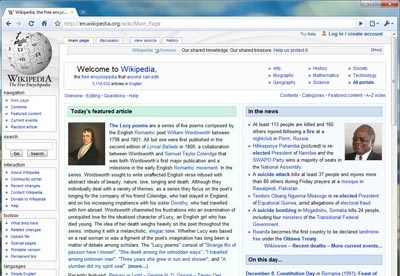The image depicts the main page of Wikipedia, rendered in a vintage format indicative of an older style of the website. The webpage is being viewed through an outdated version of Internet Explorer, which is evident from the layout of the browser's interface.

In the top left corner of the page, the well-known Wikipedia logo is prominently displayed. Adjacent to the logo, on the left side of the page, various navigation menus are lined up vertically. These menus also extend to the bottom left and far bottom left of the screen, though their specific contents are not discernible.

At the center of the page, under a green banner that reads "Today's featured article," there is an oil painting of an older white man with brown hair. The caption and details accompanying the image are too small to be read clearly, but the initial text displayed is red. Mixed in with this red text is a blue hyperlink that appears to reference "The Lucy poems."

To the right of the featured article section, there's a segment titled "In the news," which includes a photograph of an older, bald black man wearing a suit and sunglasses, smiling. The exact details of the accompanying text are too fine to be legible.

Further down the page, under "On this day," the date "December 6" is mentioned, marking "Constitution Day of Romania." There is also a partially visible reference to a feast day, although the complete name is cut off.

A vertical scrollbar is visible on the far-right side of the browser window, which is positioned at the top, suggesting that the page hasn't been scrolled down. The search bar at the top partially shows the web address: en.wikipedia.org/wiki/Main_Page, indicating the specific URL of the Wikipedia main page. The overall text on the page is quite small, making finer details difficult to ascertain.